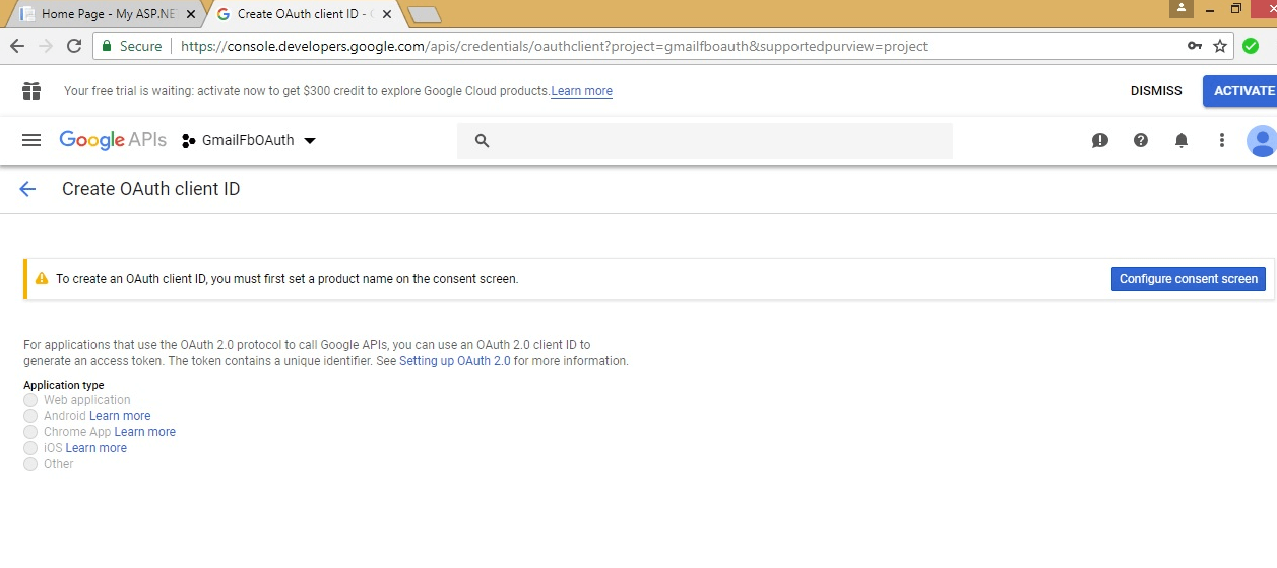The image depicts a Chrome web page with two browser tabs open. The tab on the left is labeled as the "Fullscreen Map" homepage with the URL myasp.ne, while the visible tab shows the Google Cloud console at console.developer.google.com. In this active tab, the headline reads “Create OAuth client ID,” and beneath it, there's a prominently displayed information box.

The top of the information box announces, "Your free trial is waiting: Activate now to get $300 credit to explore Google Cloud products," followed by a blue hyperlink labeled "learn more," and two action buttons: a gray "Dismiss" button and a blue "Activate" button. Below this, the page details the steps involved in creating an OAuth client ID, starting with the need to set a product name on the consent screen. The text explains that for applications utilizing the OAuth 2.0 protocol to interact with Google APIs, an OAuth 2.0 client ID is required to generate an access token, which contains a unique identifier. Further instructions can be found linked under "See setting up OAuth 2.0 for more information." The bottom right of the information box features a blue button labeled "Configure consent screen."